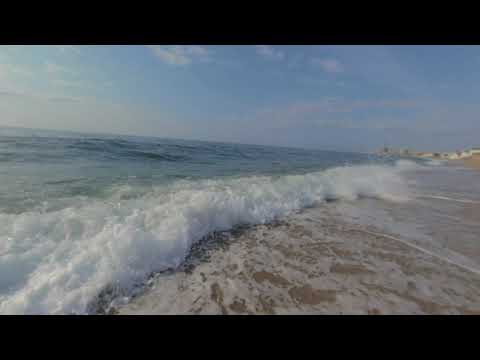This captivating beach photograph showcases a serene and natural coastal scene. The image prominently features a close-up view of a wave crashing onto the shore, creating thick, white foamy water that extends over the sand. While a little sandy texture can be seen poking through, the majority of the foreground is covered in the white foam resulting from the wave's impact. The water near the shore exhibits a gradient of blue hues, transitioning from a turquoise shade to a deeper blue as it recedes into the distance.

The sky, occupying the top third of the image, is a light blue with faint white clouds spread minimally across it, emphasizing the sunny, clear weather. There are no visible people or man-made structures prominently portrayed in the scene, maintaining a focus on the natural beauty of the beach environment. In the very bright middle of the image, there are faint, possibly blurry outlines that might hint at distant buildings, but they are not clearly defined, allowing the eye to primarily appreciate the tranquility and simplicity of the seaside. The overall perspective places you right at the water's edge, capturing a moment of pure coastal splendor.